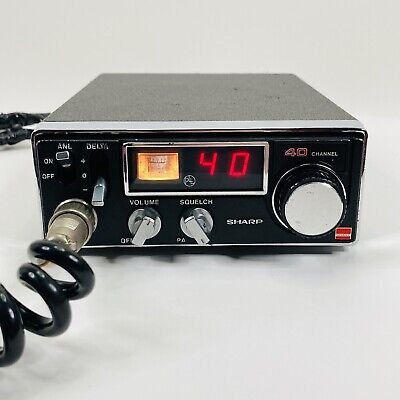The image features a small, rectangular-shaped vintage CB radio, likely from the 60s or 70s, set against a white background. The front panel is predominantly black plastic with a silver-chrome finish on the dials, giving it a sleek and shiny appearance. At the center top of the face, an illuminated red digital display prominently shows the number "40." Directly below the display are two metal-looking, flat knobs labeled for "Volume" and "Squelch." To the right, there is a larger dial encased in a plastic ring, marked "40 Channel" above it. The lower left section houses a port with a coiled black wire extending out, connecting to what would be the handheld microphone. There are additional switches on the panel for display and delay functions. The overall condition suggests it is well-preserved and might appeal to collectors on platforms like Etsy or eBay. The back section appears gray, indicating it was designed to be installed in or under a vehicle's dashboard. The unit is labeled as being manufactured by Sharp, underscoring its authenticity and period-specific design.